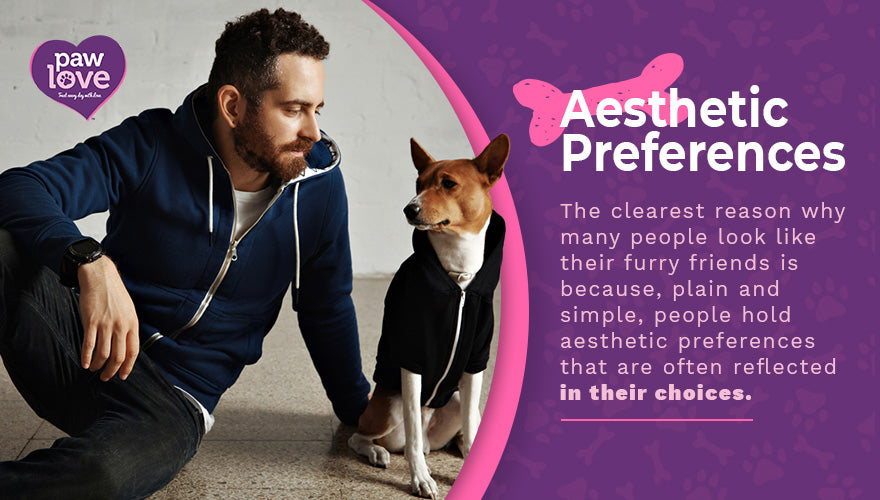The advertisement is divided into two distinct sections. On the left side, a white man with curly brown hair, an orange mustache, and beard is seen sitting on the floor, propped up by his right arm. He wears a blue zip-up sweatshirt with white strings and blue slacks. Next to him, a medium-sized dog with pointy ears, a tan face, sharp features, and a white body sits upright, also wearing a matching blue zip-up hooded sweatshirt. Both the man and the dog are looking at each other.

The right half of the ad features a purple background with a pink dog bone at the top. Inside the dog bone, white text reads "AESTHETIC PREFERENCES." Below this is a paragraph in pink text explaining that "the clearest reason why many people look like their furry friends is because, plain and simple, people hold aesthetic preferences that are often reflected in their choices." In small print, the name "Paul Love" appears, suggesting an association with a charitable organization.